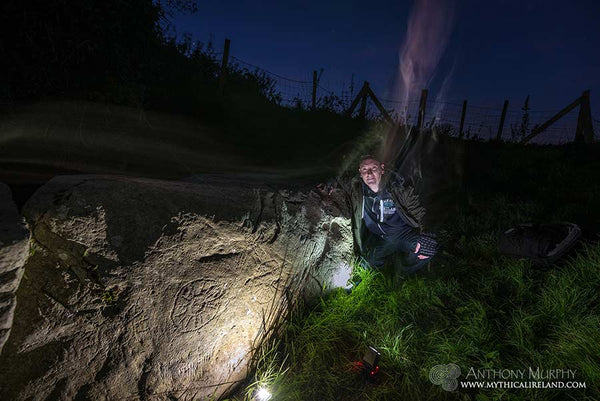In this evocative nighttime scene, the photograph, credited to Anthony Murphy from www.mythicalireland.com, captures a mysterious and somber atmosphere. A field stretches into the distance, shrouded in darkness, with faint wisps of smoke rising into the starlit sky. The silhouettes of trees and bushes form an eerie background. In the foreground, a man dressed in dark clothing—comprising a jacket, pants, and shirt—squats beside an enormous, mythical creature. The beast, resembling a dragon, lies on the ground with its massive, gray-colored body and distinctively large head and feet. Notable markings, including a pattern on its side that features a large round emblem with intricate designs, add to the enigmatic allure of the scene.